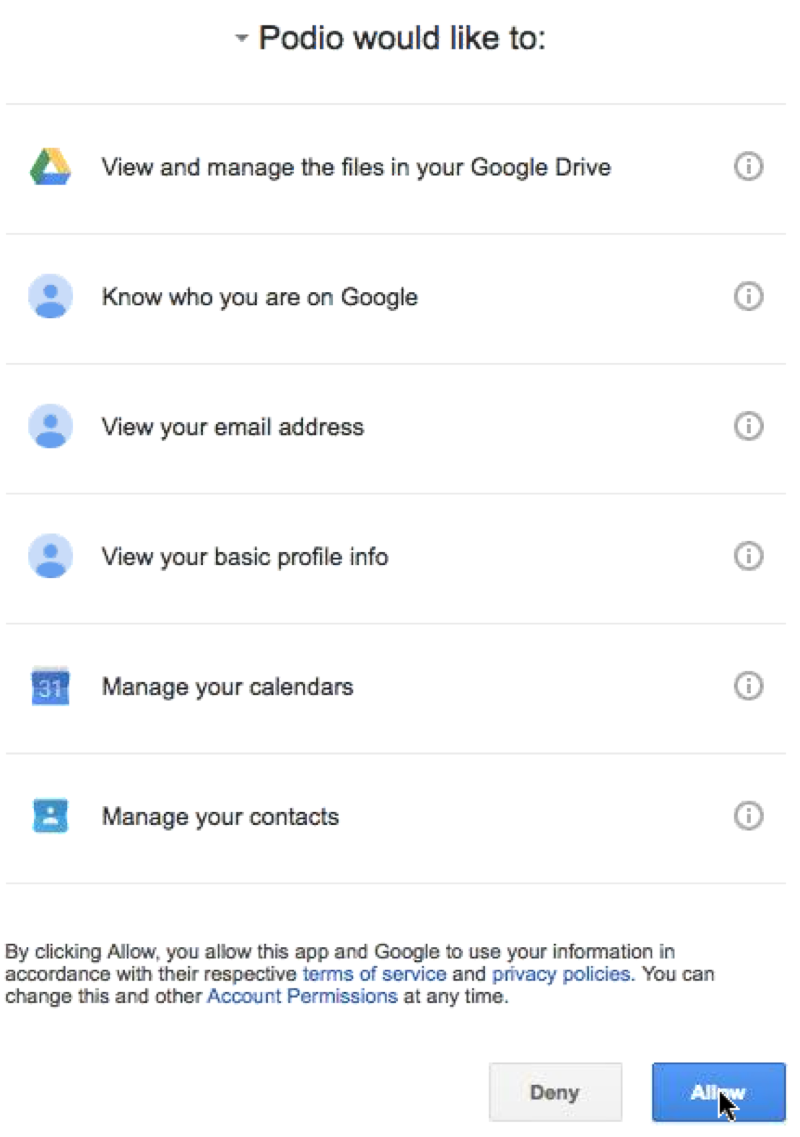A screenshot capturing a Google authorization request window with a clean white background and centered black text at the top. On the left, a small grey dropdown arrow precedes the text "Poto would like to." Below the heading, various permissions are listed alongside colorful icons: a green, yellow, and blue triangle icon representing Google Drive, next to the text "View and manage your files in Google Drive." This is followed by a light blue icon with a darker blue figure and text stating "Know who you are on Google." Similarly styled icons and text continue, detailing permissions such as "View your email address," "View your basic profile," "Manage your calendars," and "Manage your contacts." Each permission line includes a circular icon with the letter 'i' on the right side for more information. At the bottom of the window, there is a disclaimer about data usage: "By clicking 'Allow,' you permit this app and Google to use your information in accordance with their respective terms of service and privacy policies. You can change these and other account permissions at any time." Below this disclaimer, a blue "Allow" button is highlighted, with a black arrow indicating an imminent click.